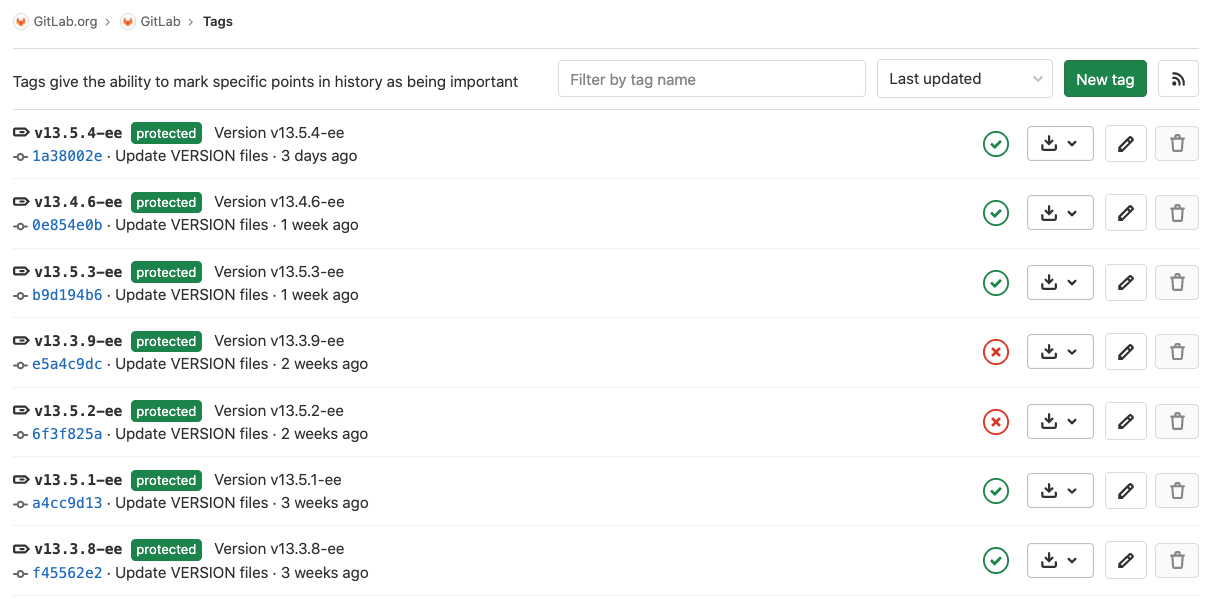The image depicts a detailed view of the "Tags" section within a GitLab repository interface. Here's the restructured detailed caption:

---

The screenshot shows the "Tags" section of a GitLab repository with a white background. In the upper left-hand corner, the navigation path is displayed. It begins with a white circle containing a red, downward-pointing arrow followed by the URL "gitlab.org" (with "Git" and "Lab" capitalized). A gray arrow points to the right indicating navigation into the "gitlab" section (similarly capitalized). Another white circle with a red arrow is followed by the label "tags" (capitalized as "TAGS") in black text.

A description below the navigation path reads: "Tags give the ability to mark specific points in history as being important."

To the right of this description, there is a white search box with gray placeholder text that reads, "Filter by tag name." Further right is another box that displays "Last updated" in black text alongside a downward arrow for sorting options. Adjacent to this, a green button with white text reads, "New tag." Next to this button appears a box icon with a Wi-Fi signal symbol, suggesting additional data settings or connectivity options.

Below these navigation and filter options, detailed information about specific tags is presented:

1. **Tag V13.5.4-EE**
   - **Protected version:** V13.5.4-EE
   - **Commit ID:** 1838002E (in blue text)
   - **Status:** Update version files three days ago
   - **Icons:** Green check mark, download icon, pencil icon, trash can icon

2. **Tag V13.5.3-EE**
   - **Protected version:** V13.5.3-EE
   - **Commit ID:** B9D194B6 (in blue text)
   - **Status:** Update version files one week ago
   - **Icons:** Green check mark, download icon, pencil icon, trash can icon

3. **Tag V13.5.1-EE**
   - **Protected version:** V13.5.1-EE
   - **Commit ID:** A4CC9D13 (in blue text)
   - **Status:** Update version files three weeks ago
   - **Icons:** Green check mark, download icon, pencil icon, trash can icon

4. **Tag V13.5.2-EE**
   - **Protected version:** V13.5.2-EE
   - **Commit ID:** 6F3F825A (in blue text)
   - **Status:** Update version files two weeks ago
   - **Icons:** Red X, download icon, pencil icon, trash can icon

5. **Tag V13.4.6-EE**
   - **Protected version:** V13.4.6-EE
   - **Commit ID:** 0E854E0B (in blue text)
   - **Status:** Update version files one week ago
   - **Icons:** Green check mark, download icon, pencil icon, trash can icon

6. **Tag V13.3.9-EE**
   - **Protected version:** V13.3.9-EE
   - **Commit ID:** E5A4C9DC (in blue text)
   - **Status:** Update version files two weeks ago
   - **Icons:** Red X, download icon, pencil icon, trash can icon

7. **Tag V13.3.8-EE**
   - **Protected version:** V13.3.8-EE
   - **Commit ID:** F45562E2 (in blue text)
   - **Status:** Update version files three weeks ago
   - **Icons:** Green check mark, download icon, pencil icon, trash can icon

Each tag entry includes a commit identifier in blue text, timestamp information in black text, and a series of icons for additional actions such as download, edit, or delete. Some entries feature a green outlined circle with a check mark indicating successful updates, while others have a red outlined circle with an X indicating possible issues.

---